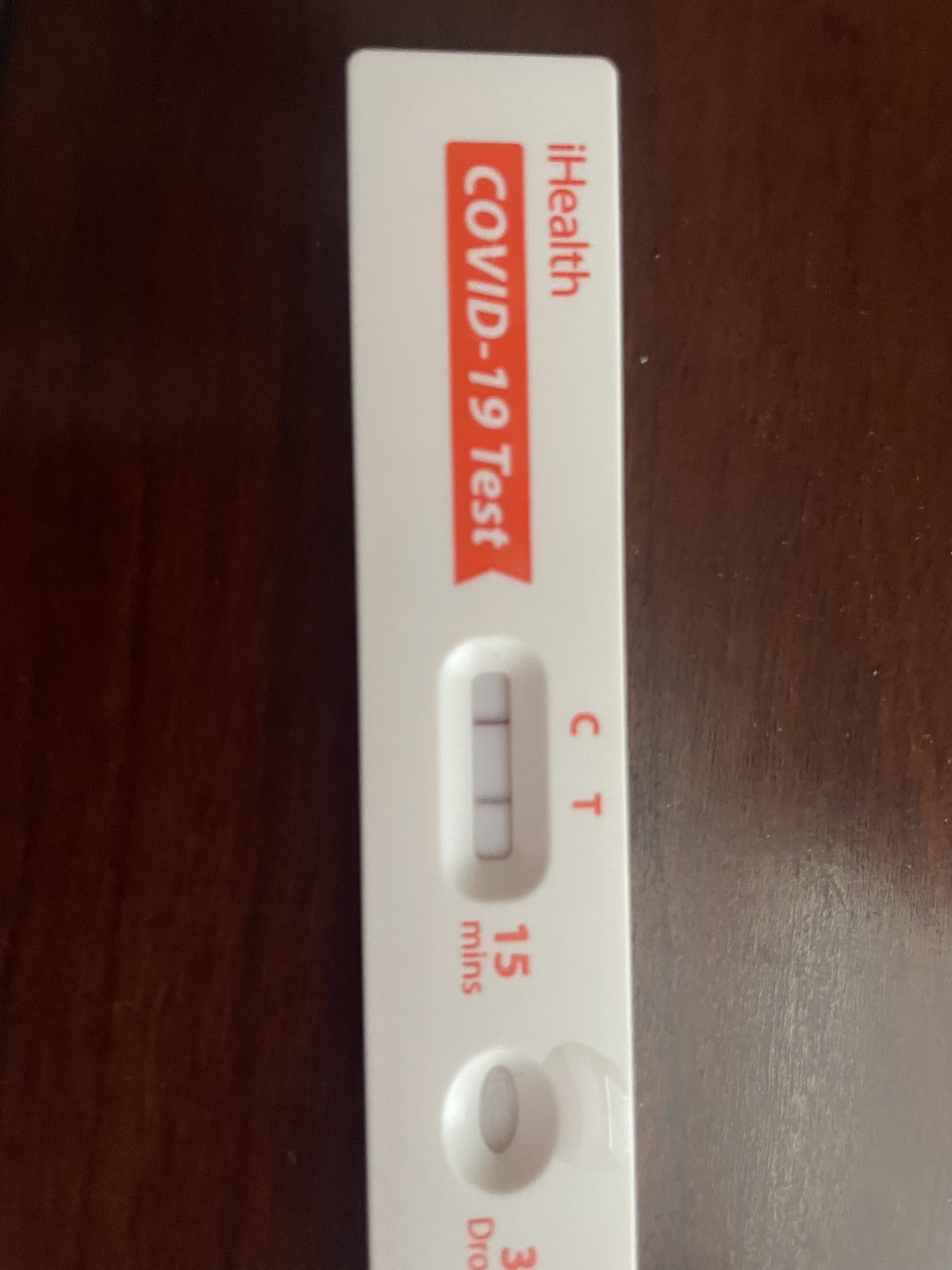A close-up image of a COVID-19 rapid test kit displayed vertically on a brown wooden tabletop. At the top of the test stick, in red text horizontally, it reads "Eye Health." Below that, in a white font within a red banner, it states "COVID-19 Test." To the right, there is a small circular window with a white center and two black lines. Above this window, the text "CT" is visible. Next to the circular window, it says "15 mins" indicating the test duration. Below this is another oval-shaped window. Near the bottom, partial text can be seen, saying "3 DRO..." due to the image being cut off. Light reflects off the bottom right corner of the tabletop, adding a subtle highlight to the scene.